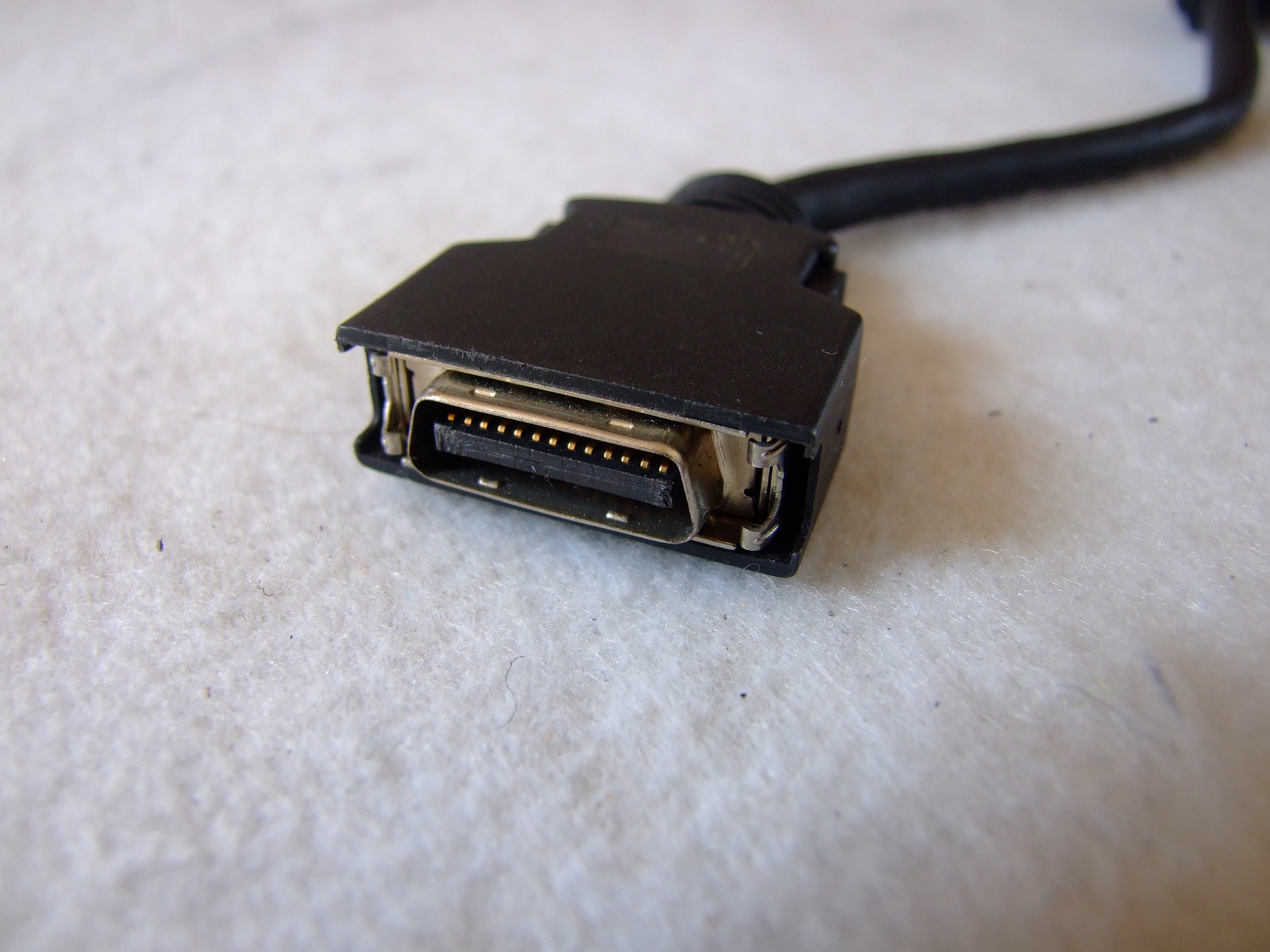The image depicts a vintage black cable likely used for connecting old computer equipment, such as a printer or potentially a monitor, to a desktop computer. The cable features gold connectors inside a silver outer casing at the connection point, with a rectangular black plastic or metal piece encasing this end. Approximately 10 to 15 gold connector pins are visible within the port. The black cable extends diagonally from the middle of the photo upward and to the right, disappearing out of the frame. It rests on a white felt-like fabric, possibly a blanket or pillow, which has a few scattered black dust particles on its surface.